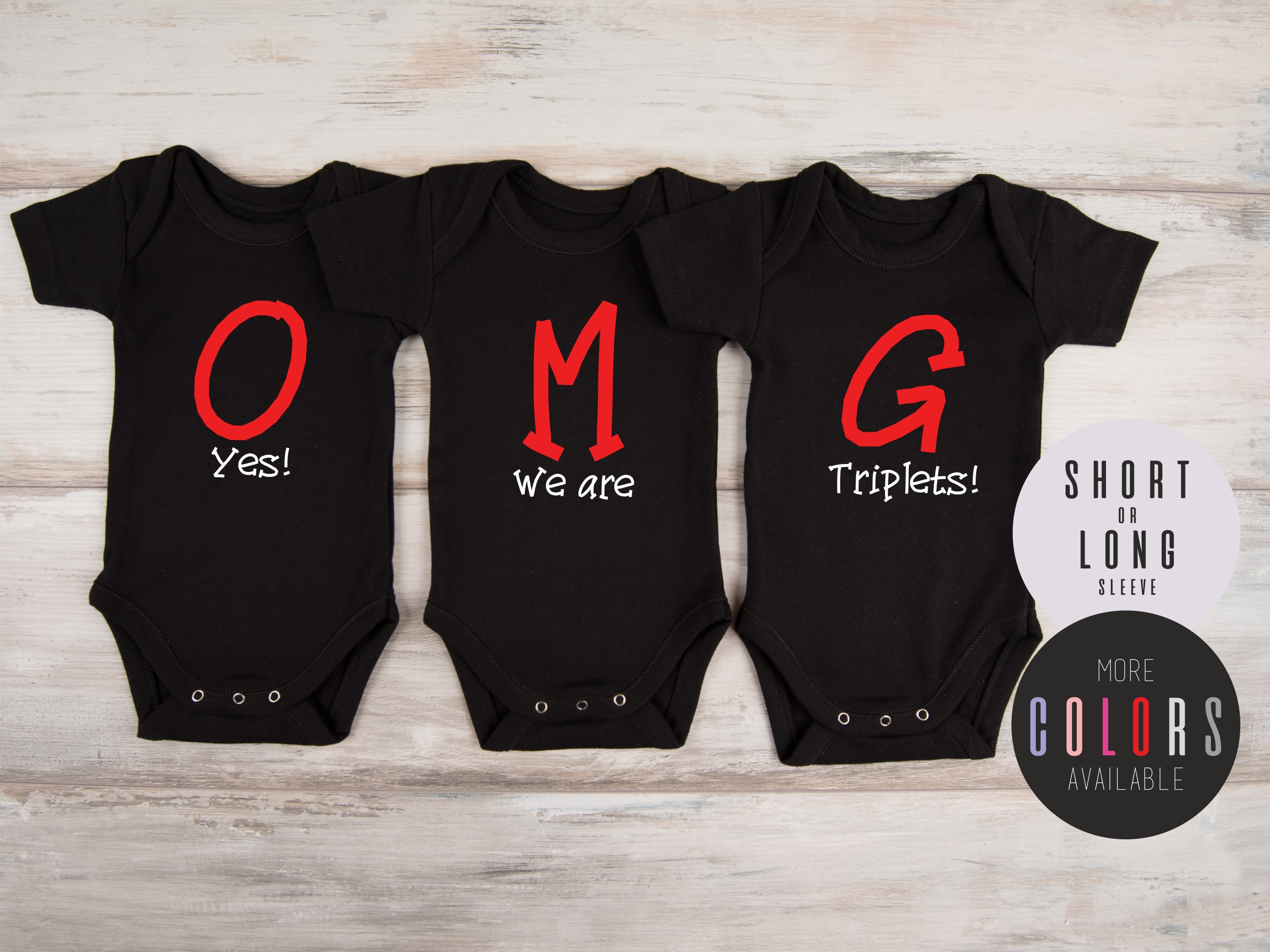This image showcases a coordinated set of three black newborn onesies laid out side by side on a pale wooden table. Each onesie bears a bold red letter prominently above a white word or phrase, forming a sequential message when viewed together. The first onesie features a large red "O" with "yes!" in white below it. The second has a red "M" with "we are" in white text. The third onesie displays a red "G" with "triplets!" in white. Collectively, they spell out "OMG yes! we are triplets!" The onesies are short-sleeved and designed with typical three-snap closures at the crotch. In the top right corner, a gray circle indicates that both short and long sleeve versions are available, and a black circle notes that more color options are offered. The onesies are arranged with their shoulders touching, highlighting their unity as a set.